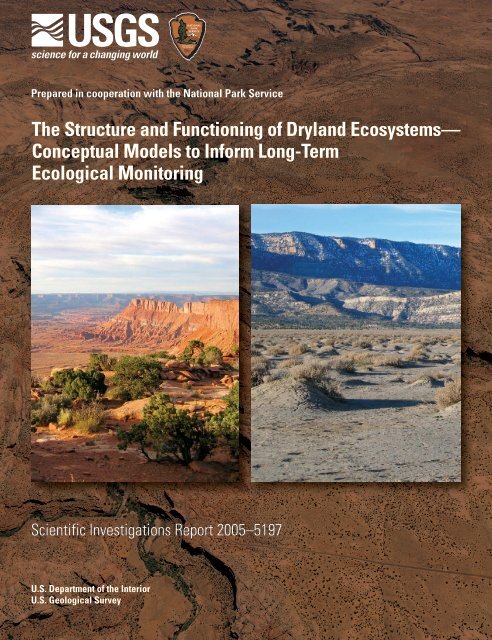This detailed aerial photograph, used as a cover for a scientific journal or report, showcases a desert landscape in a light red to dark brown gradient with a prominent vertical gorge at its center. Overlaid on this image are two smaller photographs: the left one features striking red rock formations with scattered green trees under a cloudy white sky, while the right one displays a more subdued brownish-gray desert scene with tufts of grass, distant gray and white rock formations, pale green trees, and a clear blue sky.

In the upper left corner, there is a white logo with a black band, labeled "USGS Science for a Changing World," accompanied by the iconic National Park Service arrowhead badge. The text also indicates the collaboration with the National Park Service by stating "prepared in cooperation with the National Park Service."

Above the two central photographs, the text "The Structure and Functioning of Dry Land Ecosystems: Conceptual Models to Inform Long-Term Ecological Monitoring" is prominently displayed. Beneath the images, the designation "Scientific Investigations Report 2005-5197" is given. At the bottom left of the frame, the affiliations "US Department of the Interior" and "US Geological Survey" are listed, further emphasizing the authoritative nature of the report.